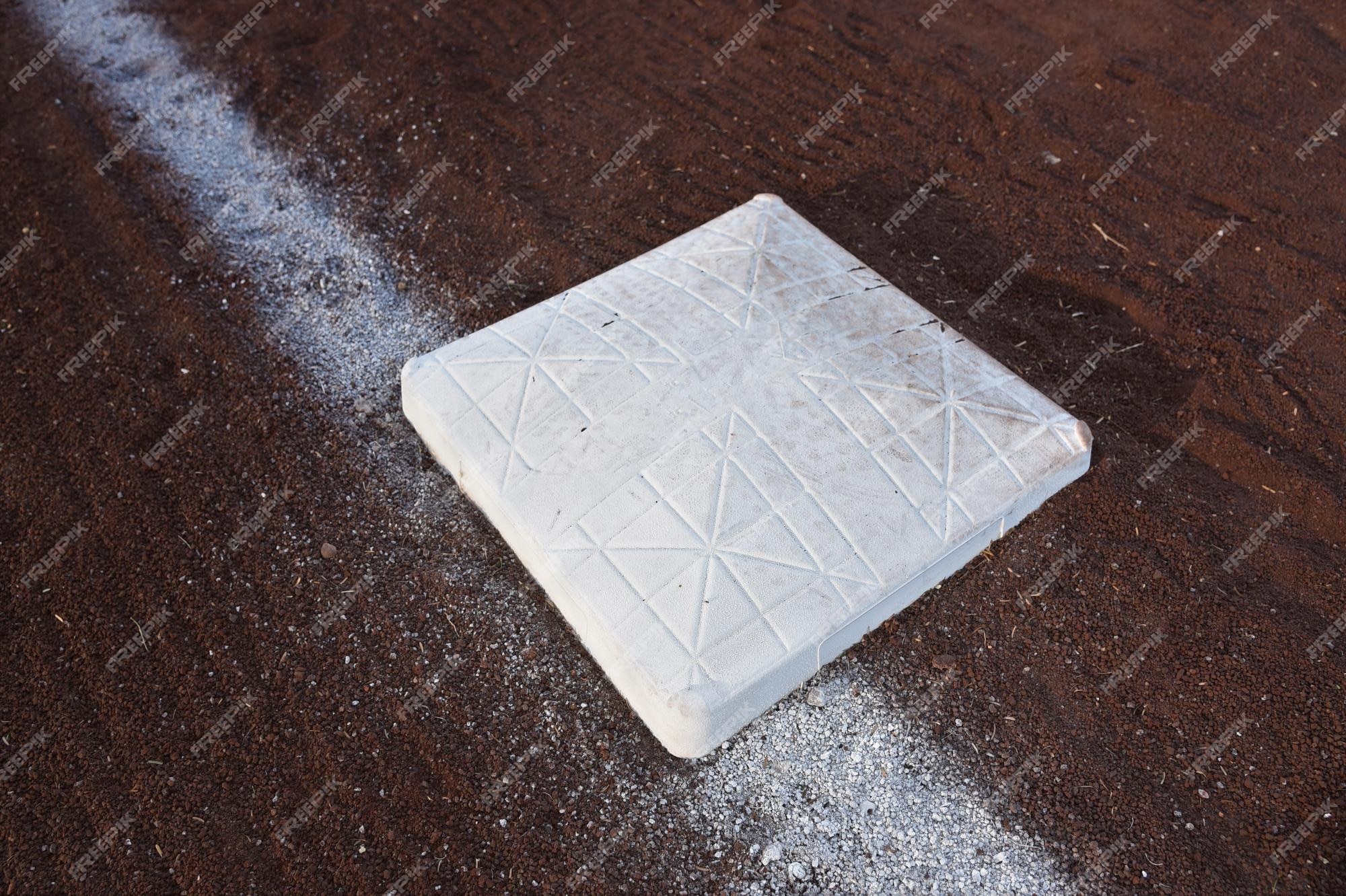The image features an up-close view of a baseball base positioned against what appears to be a dark, reddish-brown dirt background. The base itself is a white, slightly raised square, approximately a foot in length on each side and about two inches in height. The center of the base appears slightly mounded, giving it a cushiony, poofy look designed to prevent injuries during play. The surface shows signs of wear, with scuff marks and dirt highlighting its usage. Notably, the base is textured with quilted lines that form smaller squares and intersecting diagonal lines creating an 'X' pattern in each corner. A powdery white chalk line runs along the left edge and partially beneath the base, likely indicating a baseline on a baseball or softball field. An overlay of white text marking the image as "free pics" repeats diagonally across the entire image, indicating copyright.